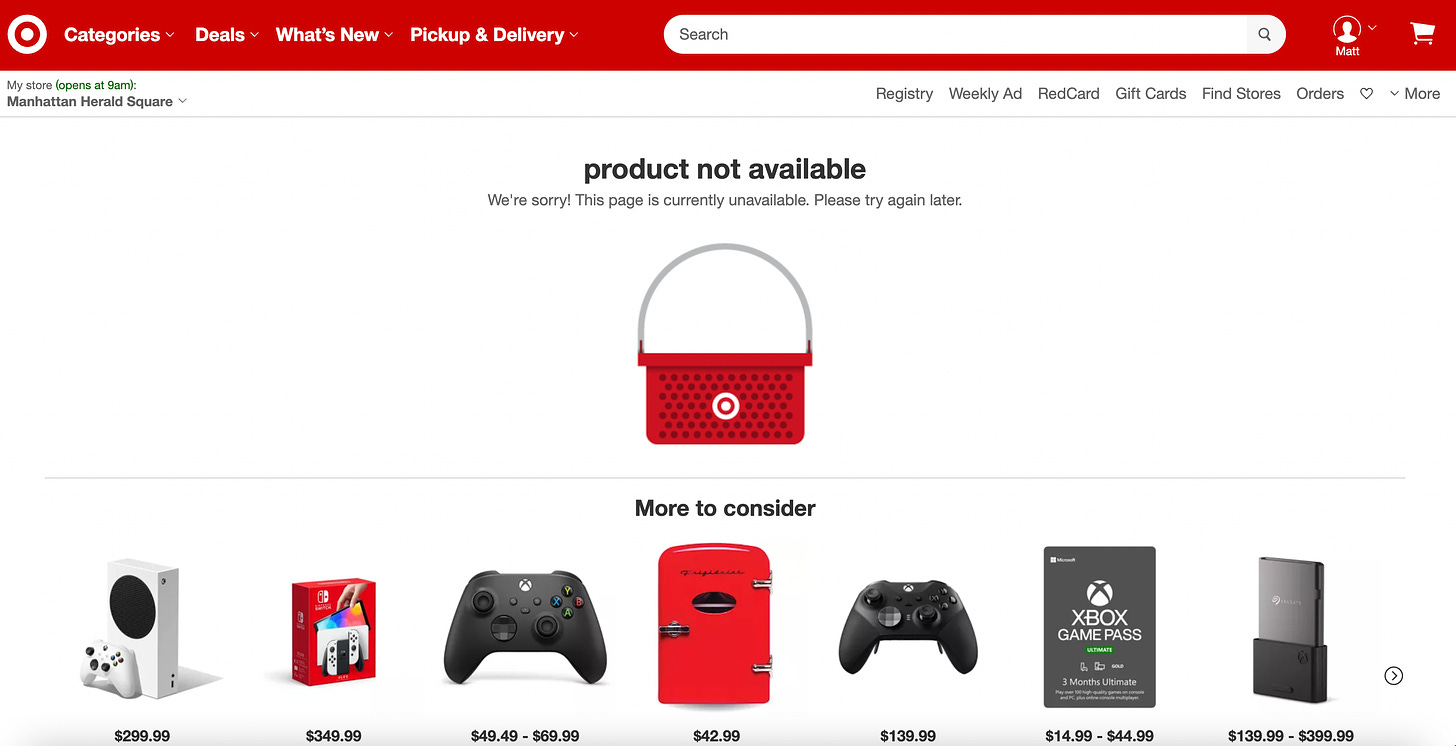This screen capture from the Target website prominently features a red banner at the top with the iconic white Target logo followed by several navigation options: "Categories," "Deals," "What's New," "Pickup & Delivery," all situated next to a white search box with a gray magnifying glass. A white circle with a down arrow and a white cart icon are present to the right. Below this, the page highlights "My Store" in green, identified as "Manhattan, Herald Square" in black text.

On the right-hand side, the options include "Registry," "Weekly Ad," "RedCard," "Gift Cards," "Find Stores," "Orders," and an icon of a heart followed by "More," all in gray text. 

The main content reveals an error message in bold black text: "Product not available," and, "We're sorry this page is currently unavailable, please try again later." Accompanying this message is a cartoon illustration of a red Target basket with a white bullseye and a gray handle.

Below, the section "More to Consider" features various product images and prices:
- A white video gaming system priced at $299.99.
- A red handheld gaming system boxed item at $349.99.
- A black game controller with blue, gold, red, and green buttons priced between $49.49 and $69.99.
- A retro 50s style red mini refrigerator costing $42.99.
- Another black game controller priced at $139.99.
- Xbox Game Pass options ranging from $14.99 to $44.99.
- A gray and silver thumb drive-like device priced between $139.99 and $399.99.